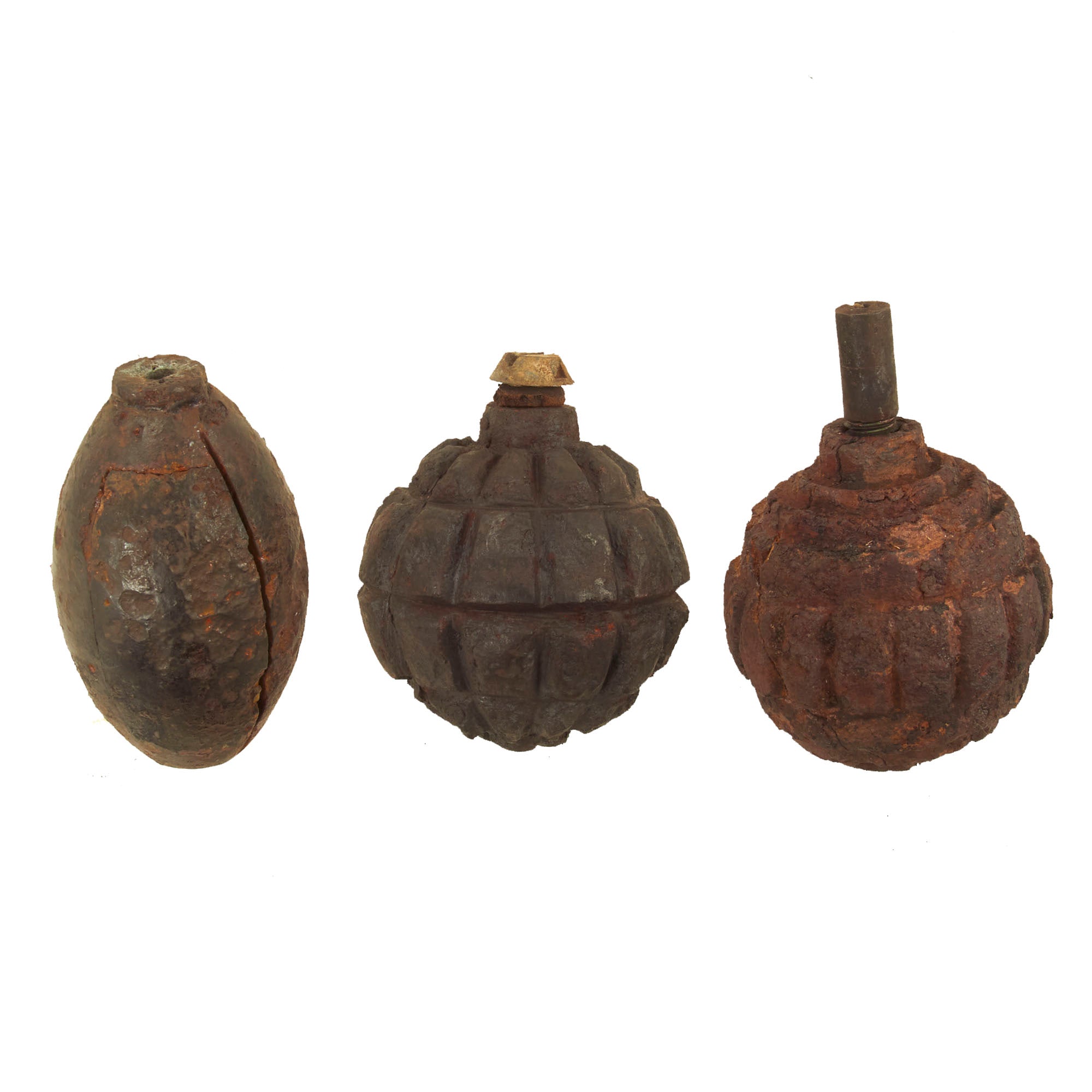The horizontal image depicts three antique hand grenades positioned upright against an uninterrupted white background, creating the illusion that they are floating in an empty white void. Each grenade varies in shape and condition, displaying distinct characteristics:

1. The grenade on the left is egg-shaped with a flat top, characterized by heavy rust and cracks. Originally black, it now has a mixture of rust and brown coloration. Unlike the others, this grenade's detonating mechanism and fuse have been removed, leaving a noticeable hole at the top.

2. The central grenade is more spherical with numerous indentations that form a pattern of small squares across its surface. It is the least rusted of the trio, bearing a brown-greenish hue. At its very top, a silver ring is visible, indicating a possible detonating mechanism.

3. The grenade on the right closely resembles the middle one in its spherical shape but is larger and has a deep reddish tint due to extensive rust. It features square cutouts similar to the middle grenade and has a prominent cylinder or pull mechanism protruding from its top.

Together, these details offer a comprehensive view of the distinct features and conditions of the three grenades, emphasizing their aged and deteriorated appearance.